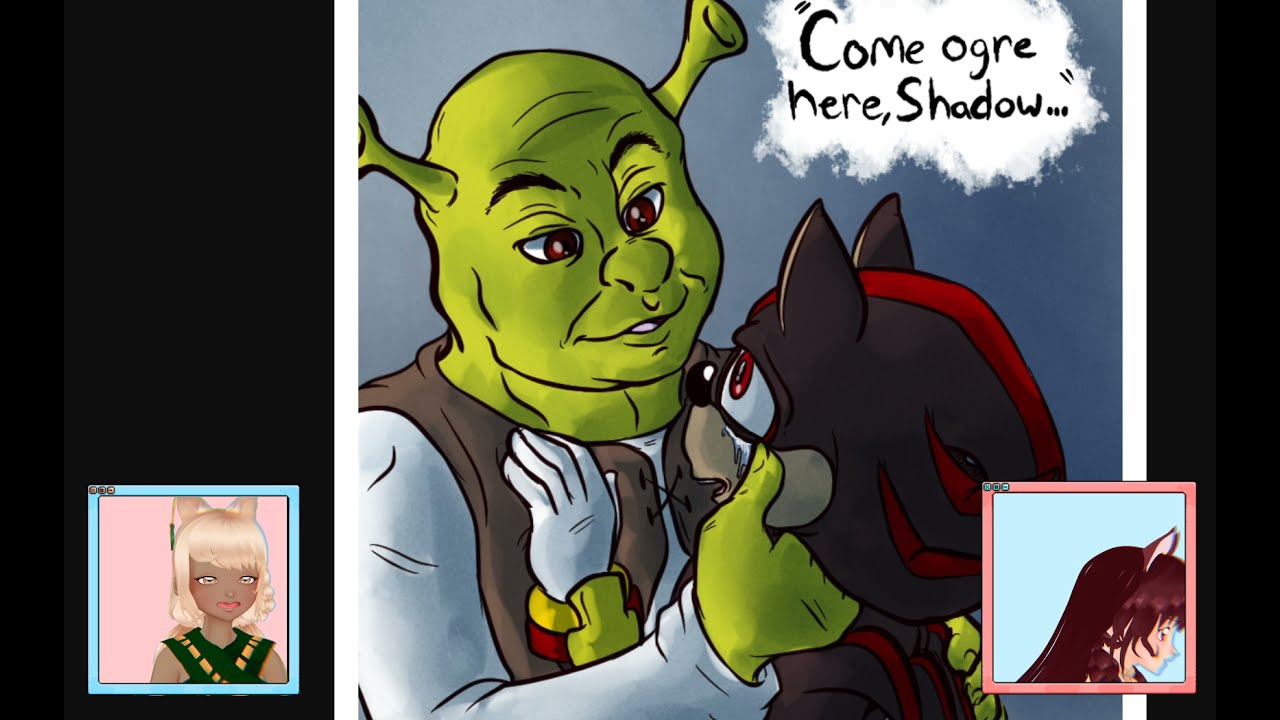The image is a screenshot from an animated cartoon or video game. Dominating the center is an amateur drawing of Shrek, a green ogre with two horns protruding from his head, dressed in a white shirt and gray vest. He is gently holding a distressed figure resembling Knuckles from the Sonic video games. Knuckles, characterized as a black and red hedgehog with white gloves and a green cuff on his left wrist, appears to be crying while looking up at Shrek. They are surrounded by a blue background with white outlines. Above them, a speech bubble resembling a white cloud of smoke contains black text that reads, "Come ogre here, Shadow."

In the lower right corner of the image, there is a smaller blue square with a pink outline featuring an anime girl with long brown hair and cat ears, depicted as walking away. Another character is situated in the lower left corner within a pink square with a blue outline, shown against a pink background. This character has brown skin, short blonde hair, and cat ears, adorned in black clothing that emphasizes a wolf-like aesthetic.